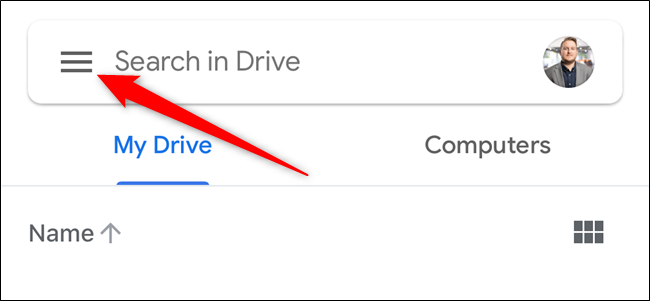The image is a detailed instructional graphic illustrating the interface of Google Drive. At the center of the graphic is a screenshot featuring the search bar at the top. To the left of the search bar is the "hamburger" icon, represented by three horizontal lines, which users can click to reveal additional menu options. Directly beneath the search bar are two tabs labeled "My Drive" and "Computers."

Further down, an arrow labeled "Name" points to a section likely indicating where file names are displayed. On the bottom right corner of the interface, there's a small icon composed of six squares arranged in two rows of three, symbolizing the grid view option for viewing files.

To the right of the search bar, there is a small avatar depicting a person in business casual attire, wearing a two-piece blazer. Overlaying the entire image is a prominent red arrow pointing directly at the hamburger icon, emphasizing that this is the focal point of the action being demonstrated.